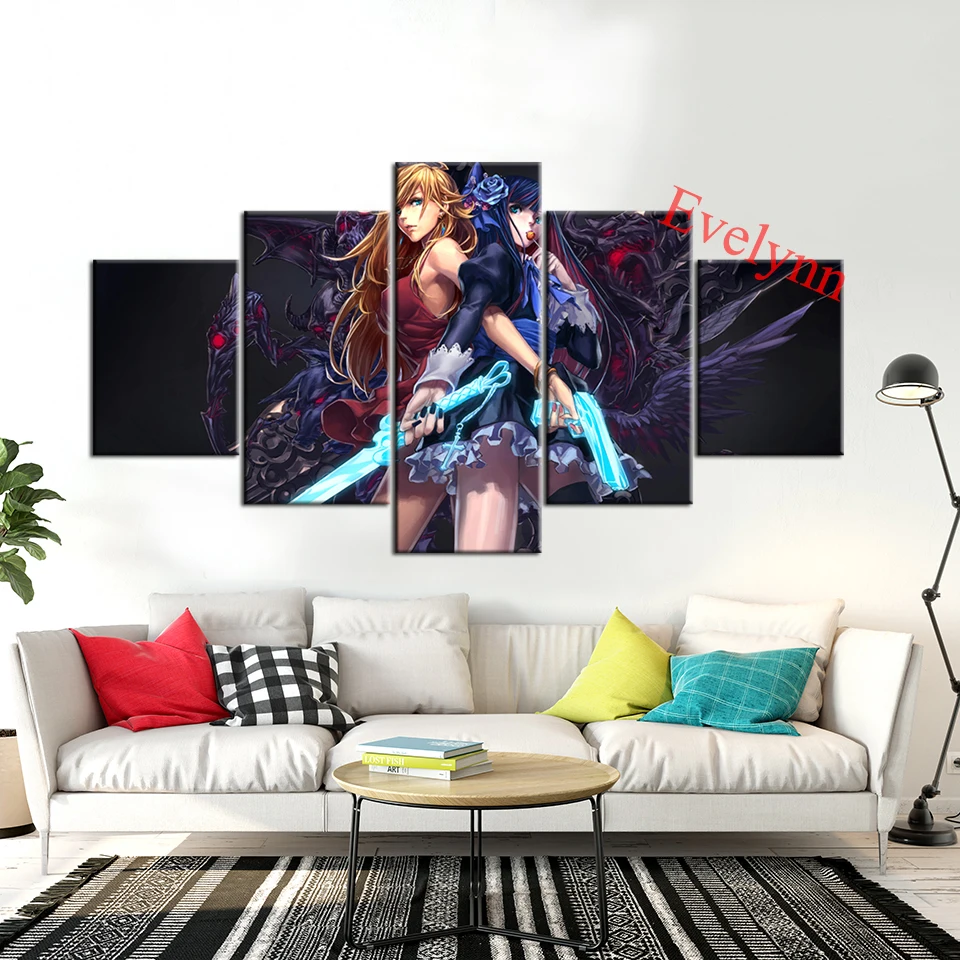The detailed image showcases a stylish living room featuring a modern white couch adorned with a variety of colorful pillows: a vibrant red pillow, a black and white checkered pillow, a bright yellow pillow, and a blue pillow with white checkmarks. In front of the couch, a round wooden coffee table with black legs holds three stacked books: a blue one, a yellow one, and a white one. This setup rests on a black and white striped rug. To the left of the couch, part of a lush green house plant is visible, while on the right, a tall black floor lamp casts a warm yellow or white light. The backdrop is a pristine white wall with a striking art arrangement. This artwork is fragmented into five separate frames, together depicting an image of two anime warrior girls: one with brown hair and a red shirt holding an icy blue gun, and the other with bluish-black hair, puffy black sleeves, and wielding a blue sword. The framed image is set against a dark backdrop with indistinct monstrous figures. Above this artwork, the name "Evelynn," spelled out in bold red letters, has been digitally added after the picture was taken.